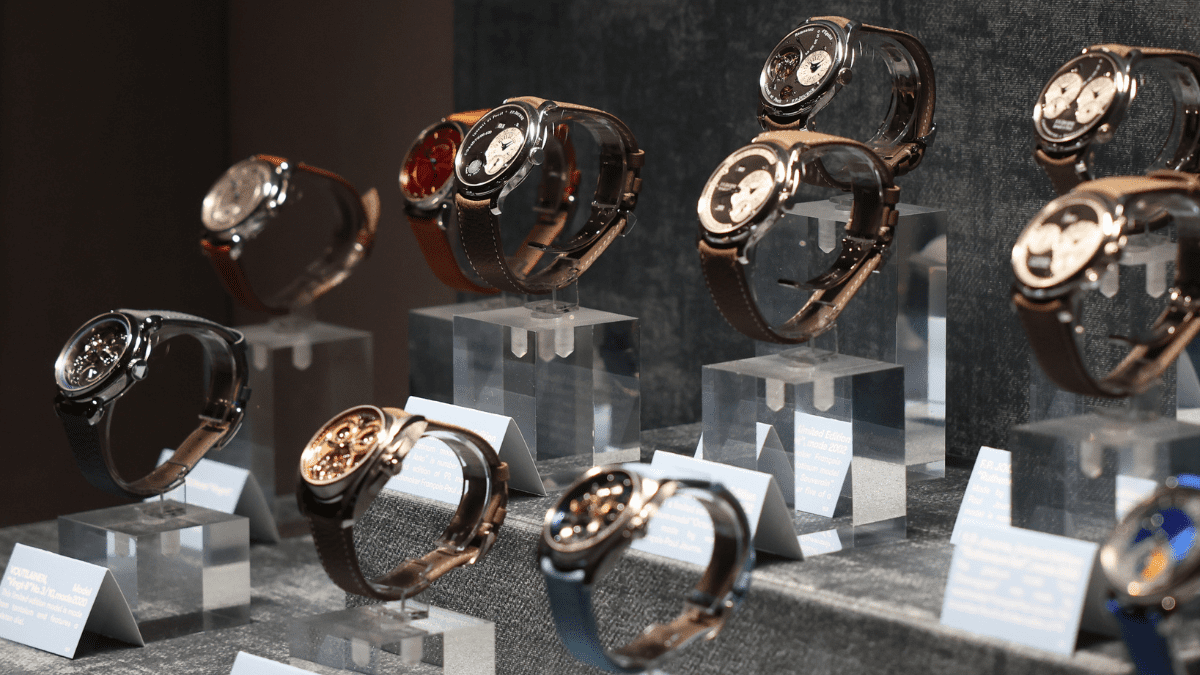The image showcases an elegant display of eleven watches, meticulously arranged on clear glass cubes against a two-toned backdrop. The back wall has a muted gray color, while the left wall is a contrasting brown. Each watch is set on its own glass pedestal, some accompanied by folded gray cards bearing white lettering that likely detail their specifications or brand.

The wristbands of the watches vary in color and material: several sport rich brown bands, a couple feature sleek black bands, and the watch positioned closest to the center boasts a distinctive gray wristband. Notably, the three watches at the bottom of the display stand out for their transparent faces, revealing intricate internal mechanisms and the mesmerizing motion of their hands.

Adding a splash of color, a watch on the left side has a striking red face. Meanwhile, other watches in the collection feature black faces with white elements, including semicircles or circles that house smaller dials, evoking the look of a stopwatch. This detailed composition not only highlights the diversity in the design and functionality of the watches but also exudes an air of sophistication and craftsmanship.